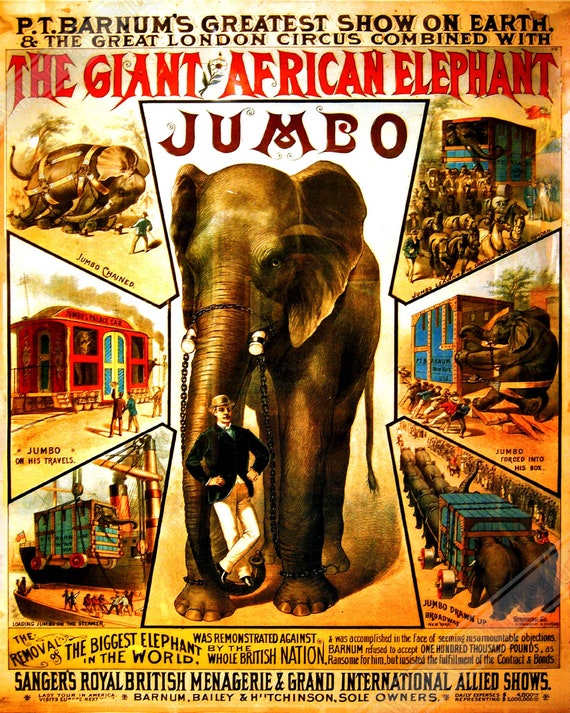This vintage-style poster is an advertisement for P.T. Barnum's Greatest Show on Earth and the Great London Circus, featuring the giant African elephant, Jumbo. Dominating the center of the poster, Jumbo is depicted in a striking bronzy goldish hue, with a bit and chain attached to his trunk and mouth, and his tusks removed. Standing atop a saddle at Jumbo's feet is a dandy-looking turn-of-the-century man, emphasizing the elephant's enormous size. Surrounding this central image, six smaller scenes illustrate the dramatic capture of Jumbo in the wild and his transportation from Africa to England by boat, train, and carriage. The top of the poster announces the show in bold black lettering with the name "Jumbo" highlighted in red. The bottom of the poster provides additional details about the showcasing of the world's largest elephant, Sanger's Royal British Menagerie, and the Grand International Allied Shows, framed by a palette of yellowish beige and brown hues that evoke the era's style.